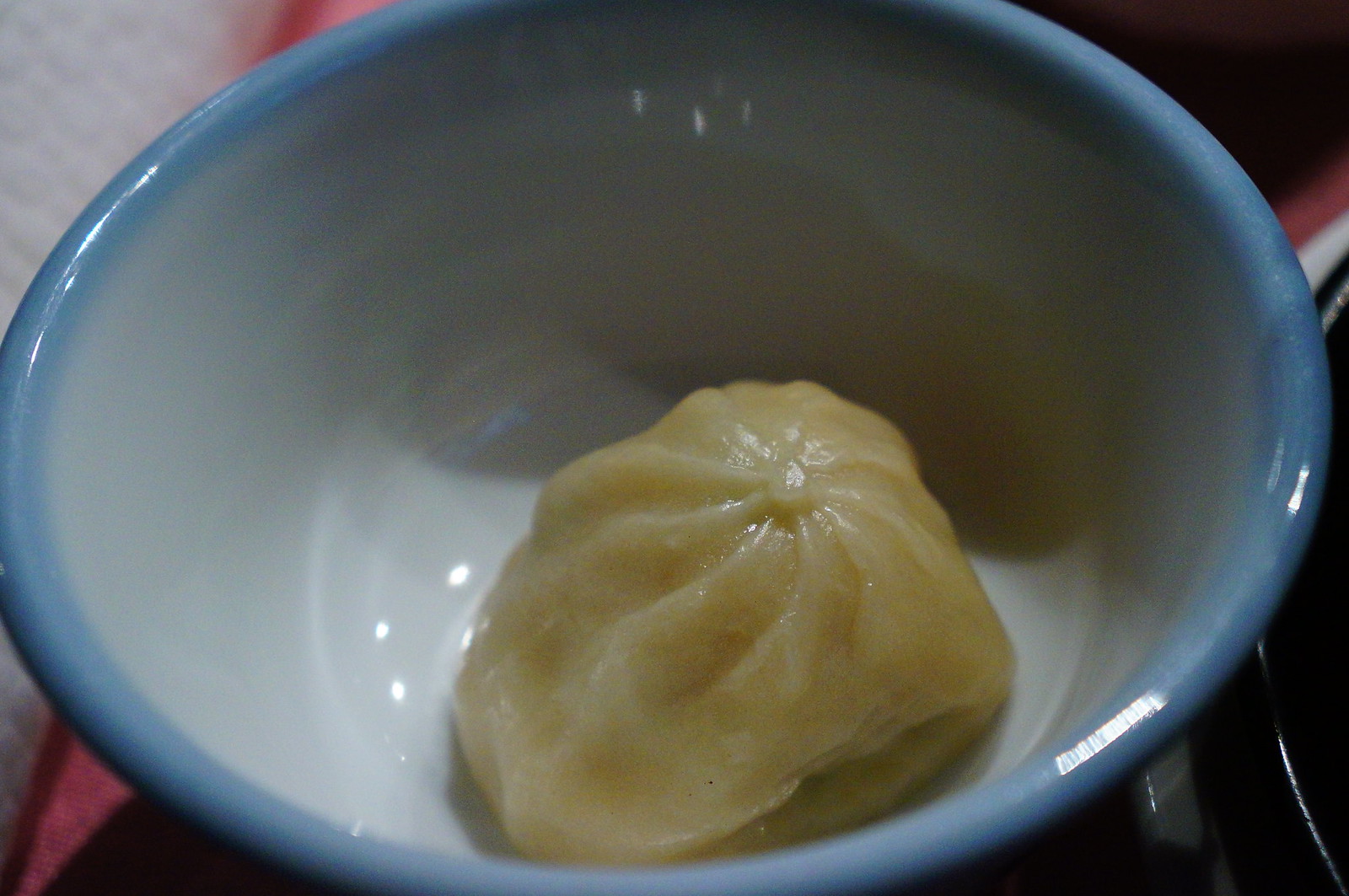In this vibrant color photograph, a single light brown, crimped dumpling rests in the bottom of a blue-rimmed bowl, positioned atop a red counter or table. The bowl's interior is a light gray hue, and it exhibits a glossy finish with noticeable reflections from both the bowl's surface and the dumpling itself, suggesting a certain dampness or moisture. Surrounding the bowl, the background is predominantly composed of alternating white and red colors, with areas of black, possibly indicating kitchenware, highlighted by silver and white outlines. The contrasting colors and reflections add depth to the image, emphasizing its culinary context.